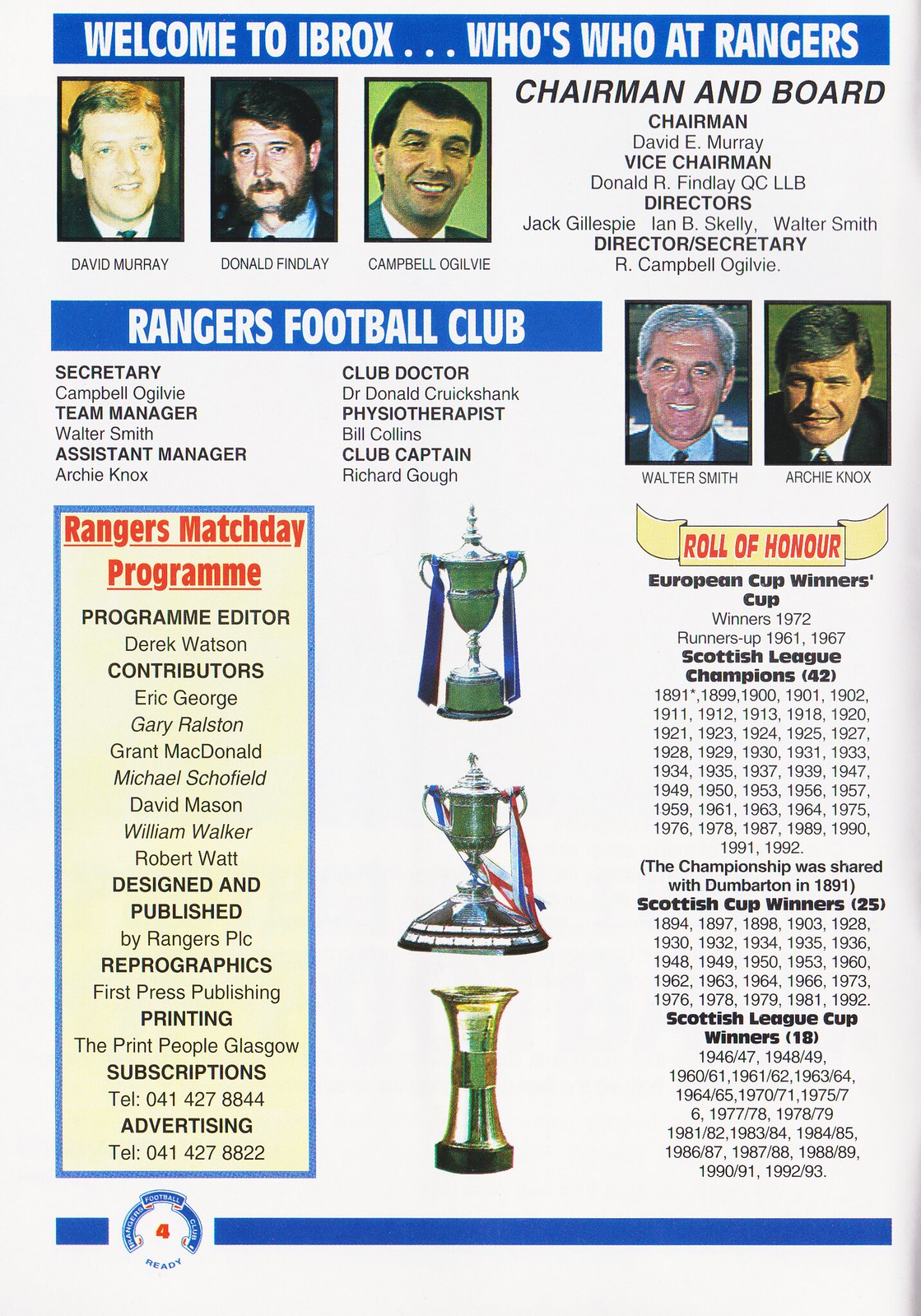This is a detailed page from a game day magazine for the Rangers Football Club in Scotland. The page features a white background with a blue rectangle across the top, containing white text that reads, "Welcome to Ibrox. Who's Who at Rangers." Below this are three profile photos on the left side, of David Murray, Donald Finlay, and Campbell Ogilvie, respectively. To the right, black text introduces the Chairman and Board: Chairman David E. Murray; Vice Chairman Donald R. Finlay, QC LLB; Directors Jack Gillespie, Ian B. Skelly, and Walter Smith; and Director/Secretary R. Campbell Ogilvie.

Another blue rectangle with white text reads, "Rangers Football Club." Below in black text are roles such as Secretary, Team Manager (Walter Smith), Assistant Manager (Archie Knox), Club Doctor, Physiotherapist, and Club Captain. To the right of this section are two more profile photos, featuring Walter Smith on the left and Archie Knox on the right.

The bottom part of the page is divided into three columns. The left column has a yellow background with a blue border, and red text at the top that reads, "Rangers Match Day Program." It lists the names of the program editor, Derek Watson, and various contributors including Eric Gorin, Rancey Gray, Grant McDonald, Michael Schufield, Dave Manson, William Walker, and Robert Walt.

In the center column, three trophies are prominently displayed. The right column is headed by a yellow banner with red text that reads, "Role of Honor," listing the club's achievements in black text: European Cup Winners Cup, Scottish League Champions, Scottish Cup Winners, and Scottish League Cup Winners.

The colors featured on the page include blue, white, green, black, brown, gray, yellow, red, gold, tan, and lime green, providing a vibrant and visually appealing layout. The entire page presents a detailed and structured overview of important personnel and accolades associated with the Rangers Football Club.